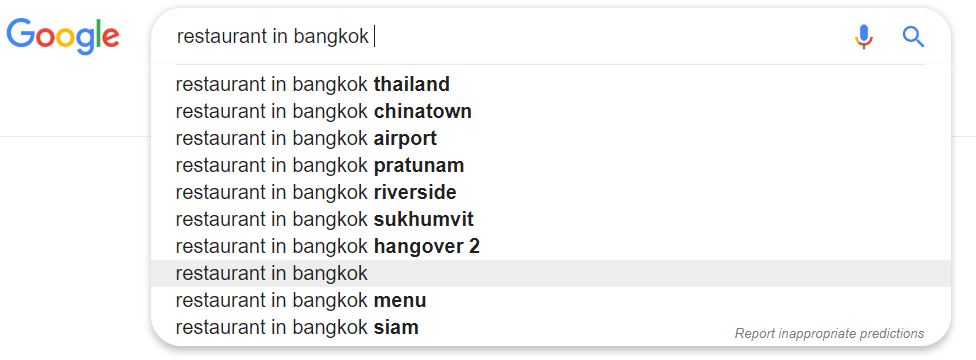This panoramic image captures a Google search interface. On the left side of the interface, the iconic Google logo is prominently displayed, consisting of a large capital 'G' in blue, followed by lowercase letters: 'o' in red, another 'o' in yellow, 'g' in blue, 'l' in green, and 'e' in red. 

In the center of the image, within the search bar, the query "restaurant in Bangkok" is typed out, with the blinking cursor placed one space after the word "Bangkok." To the right of the search bar, the blue microphone icon and a blue magnifying glass are visible.

The drop-down menu below the search bar shows several auto-suggested options, listed from top to bottom:
1. Restaurant in Bangkok, Thailand
2. Restaurant in Bangkok, Chinatown
3. Restaurant in Bangkok, airport
4. Restaurant in Bangkok, Pratunam 
5. Restaurant in Bangkok, Riverside
6. Restaurant in Bangkok, Sukhumvit
7. Restaurant in Bangkok, Hangover 2
8. Restaurant in Bangkok (this option is faintly highlighted in gray, suggesting it is currently selected or has been selected before)
9. Restaurant in Bangkok, menu
10. Restaurant in Bangkok, Siam

At the bottom right of the drop-down menu, in faint gray letters, it reads "Report inappropriate predictions."